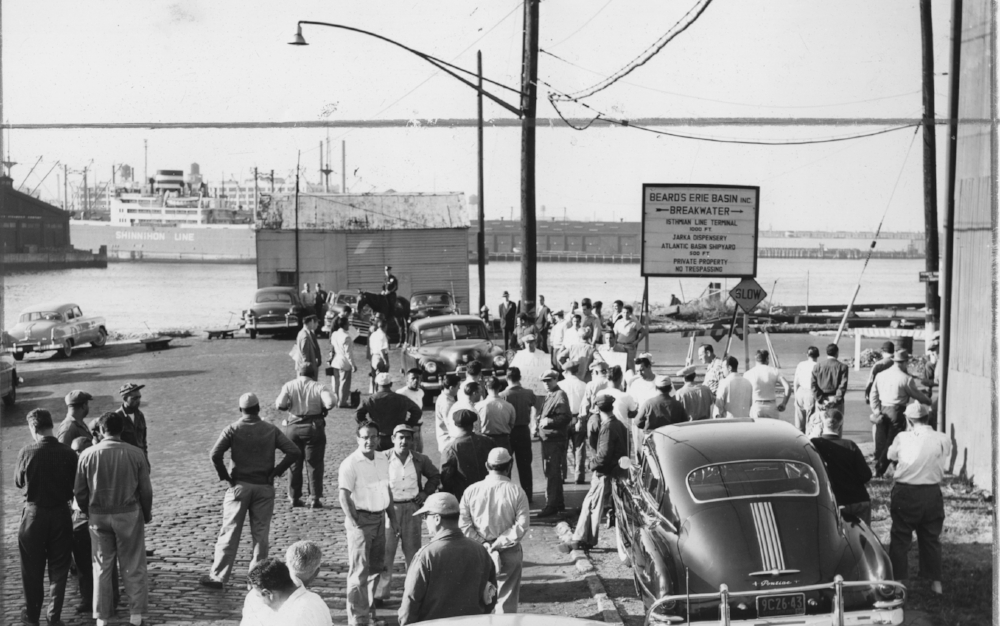This black and white vintage photograph, likely from the 1950s, depicts a bustling scene near a body of water, possibly a canal or the ocean. In the background, massive freight ships with large cabins, capable of carrying hundreds of cars and containers, are visible, indicating a busy port area. The ground is a mix of brick and cobblestone, characteristic of an old parking lot or pier.

Dozens of men, dressed in white shirts and khakis, are congregating around several sporty-looking cars from the 1950s. The men seem to be waiting for something, possibly jobs or other arrivals, though the exact context is unclear. A prominent sign in the background reads "Beards Erie Basin Inc., Breakwater, First Man Line Terminal, Jarka Dispensary, Atlantic Basin Shipyard, Private Property, No Trespassing." This suggests that the area is a significant industrial or shipyard location.

A police officer on horseback is visible in the distance, slightly out of focus, adding to the sense of a controlled yet busy environment. The sky appears gray, adding to the timeless, somber feel of the photograph. The scattered groups of men and parked cars, along with the notable signage, create a vivid snapshot of mid-20th-century industrial life near a bustling waterfront.